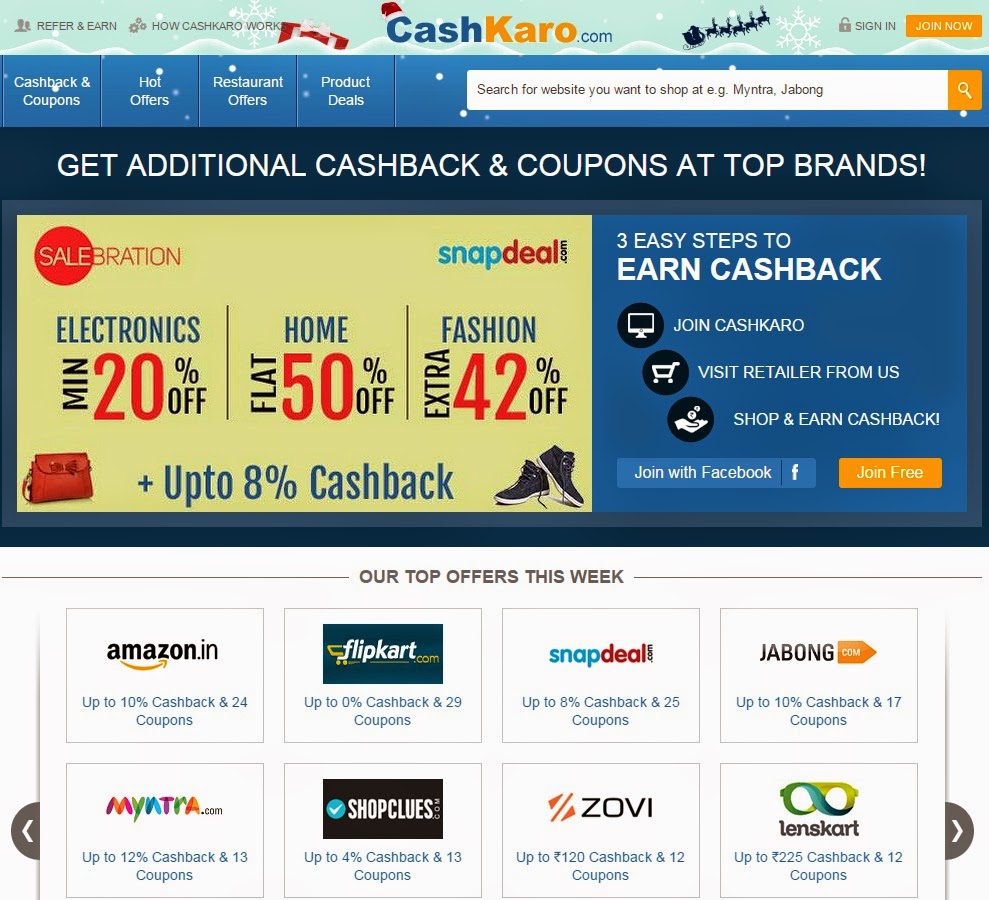Here is a descriptive caption for the provided image:

---

The screenshot displays the festive homepage of "CashKaro.com," adorned with winter holiday decorations. At the top, the site’s name "CASHKARO" is illustrated with a Santa Claus hat atop "CASH," accompanied by white snowflakes and a snowy ground effect with a partially buried red-and-white gift. The website's navigation bar includes options: "Refer and Earn," "How CashKaro Works," "Sign In," and an orange "Join Now" button. Below this, the categories "Cash Back and Coupons," "Hot Offers," "Restaurant Offers," and "Product Deals" are listed alongside a prominent search bar encouraging users to "search for a website you want to shop at," citing examples like "Myntra" and "Jabong."

The slogan "Get Additional Cash Back and Coupons at Top Brands" is followed by a promotional graphic featuring a handbag and pair of shoes. The banner reads "Sale-A-Bration," highlighting various deals on Snapdeal.com such as "Electronics, Men 20% Off," "Home, Flat 50% Off," and "Fashion, Extra 42% Off, plus up to 8% cashback." Adjacent is a guide titled "Three Easy Steps to Earn Cash Back," instructing users to "Join CashKaro," "Visit Retailer from Us," and "Shop and Earn Cash Back." Options to "Join with Facebook" via a blue button or "Join Free" via an orange button are also presented.

Below this section are thumbnails of eight web platforms labeled "Our Top Offers This Week," featuring Amazon India, Flipkart.com, Snapdeal, Jabong.com, Myntra.com, ShopClues, Zovi, and Lenskart.

---